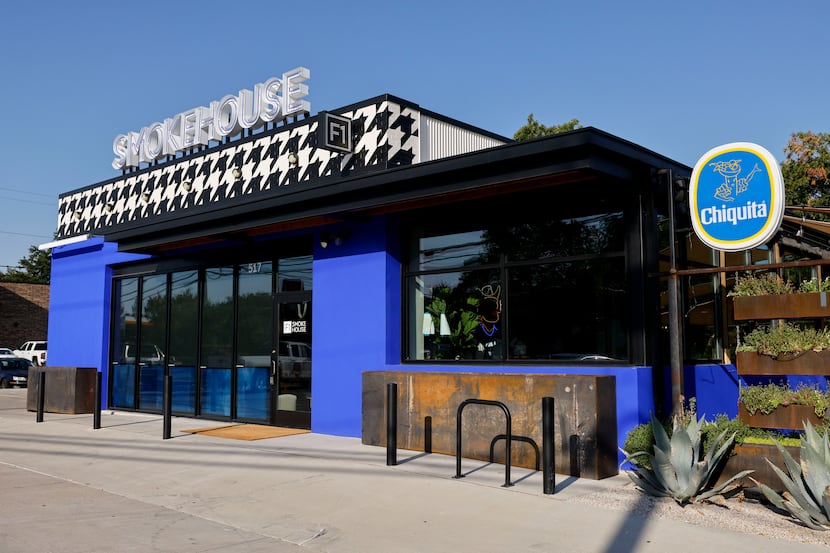In this rectangular outdoor photograph taken on a beautiful blue sky day, we see a modern-looking restaurant with a distinctive geometric design. The roof features a striking pattern in black and white, while the exterior walls are adorned with blue geometric panels and lined with sleek black-paneled windows. A black bike rack is situated on the sidewalk in the lower right corner of the image, just in front of the restaurant. Atop the roof, in bold white block letters that likely light up at night, the word "Smokehouse" is prominently displayed. In the upper right corner of the restaurant's facade, there's a large, oval-shaped sign with a blue background and a white border. The sign features the recognizable Chiquita banana logo, underscoring the restaurant's attention to eye-catching branding.